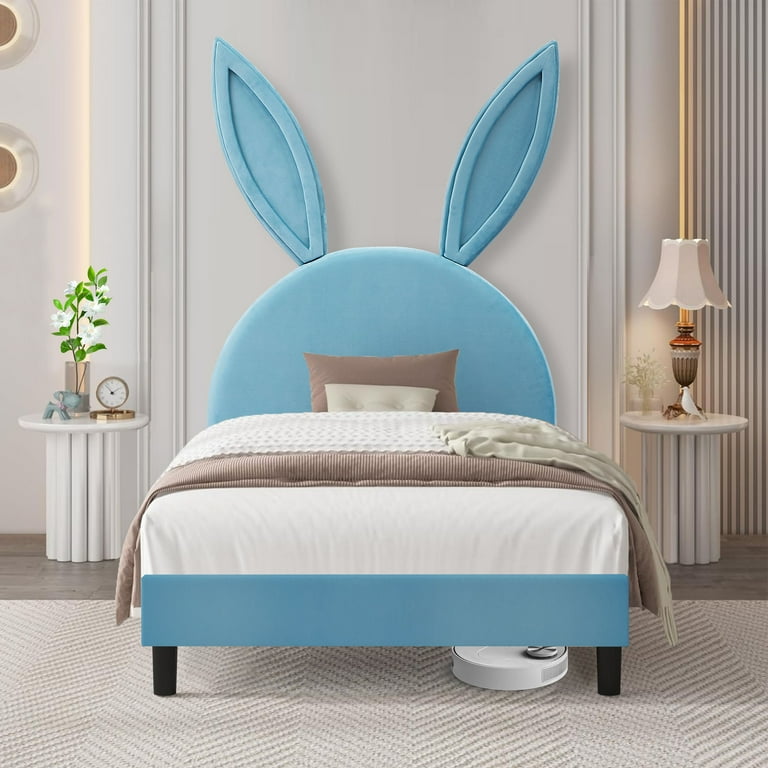The image portrays a whimsical, computer-generated bedroom centered around a large, blue bed. The bed, positioned on a white carpet covering a rustic gray hardwood floor, features a striking, blue circular headboard with two enormous bunny-like ears extending outwards, giving it a cartoony yet adult design. The bed itself has short black legs and is dressed in white sheets with a blue bed skirt. At the foot of the bed, white and brown blankets are casually layered, and a white robe hangs off the right side. The head of the bed, which rests against a light-colored wooden wall, is adorned with a gray and white pillow. 

On either side of the bed are two circular, white nightstands. The left nightstand holds a small round clock and a vase of white flowers with green leaves, while the right nightstand supports a white lamp and a small bird figurine. Above the headboard, on the top left and right of the image, faint shapes resembling half circles are partially visible on the wall. Furthermore, underneath the bed, a disc-shaped Roomba vacuum cleaner can be spotted.